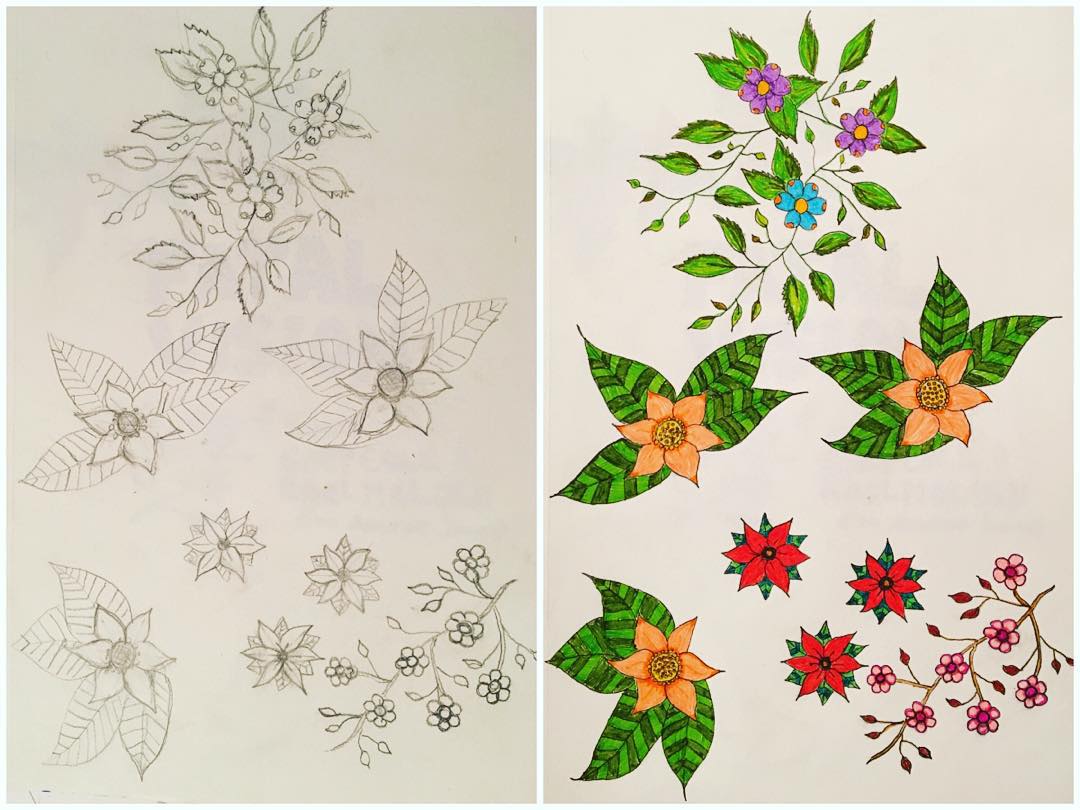The left side of the image features detailed outlines of white flowers, meticulously drawn in pencil against a plain white background. These pencil-drawn flowers are set against a stark blank canvas, providing a delicate and ethereal appearance. Interspersed among the larger flowers are smaller blooms, creating an intricate tapestry of flora. The top right corner of the image showcases a cluster of vibrant red flowers, while the bottom right corner is adorned with charming pink flowers, adding a pop of color and contrast to the monochrome left side. In the bottom left and middle sections, three radiant orange flowers emerge, providing additional warmth and balance. The right panel of the image is fully colored, serving as a vivid counterpart to the minimalist left side.